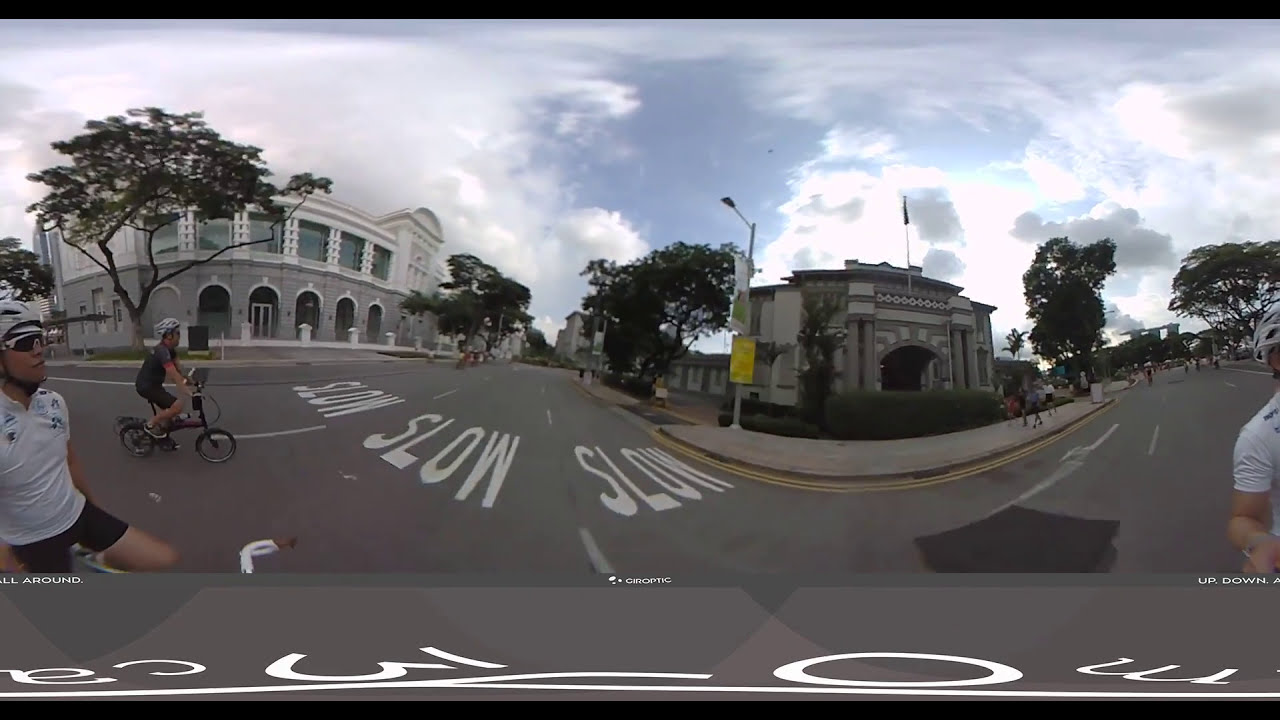The image is a panoramic, 360-degree outdoor shot capturing a city bike race during the daytime. The image features a wide black band at the top and bottom, creating a header and footer effect, with a gray band bearing the upside-down, warped text "CA 3 0 m" across the bottom inch of the photo. The photograph’s top portion displays a blue sky dotted with large white clouds. 

In the background, there are two prominent stone buildings: the one on the left is two-storied with a gray bottom and a white top featuring large arched entryways and windows, whereas the building on the right is smaller, compact, and has a single arch opening at the bottom. 

The street between the buildings is a gray road with "SLOW" painted in several lanes, and the entire scene looks warped or bubbled out in the center due to the 360-degree stitching effect typical of such panoramic images. 

In the foreground, the race participants are clearly visible. A cyclist with a white helmet, white cycling uniform, and black shorts is prominently featured towards the left, while another biker can be seen further behind. On the right edge of the image, the same cyclist in white appears again due to the panoramic effect, showing only his shoulder and helmet. A crowd is gathered on the sidewalk to the right, observing the race.